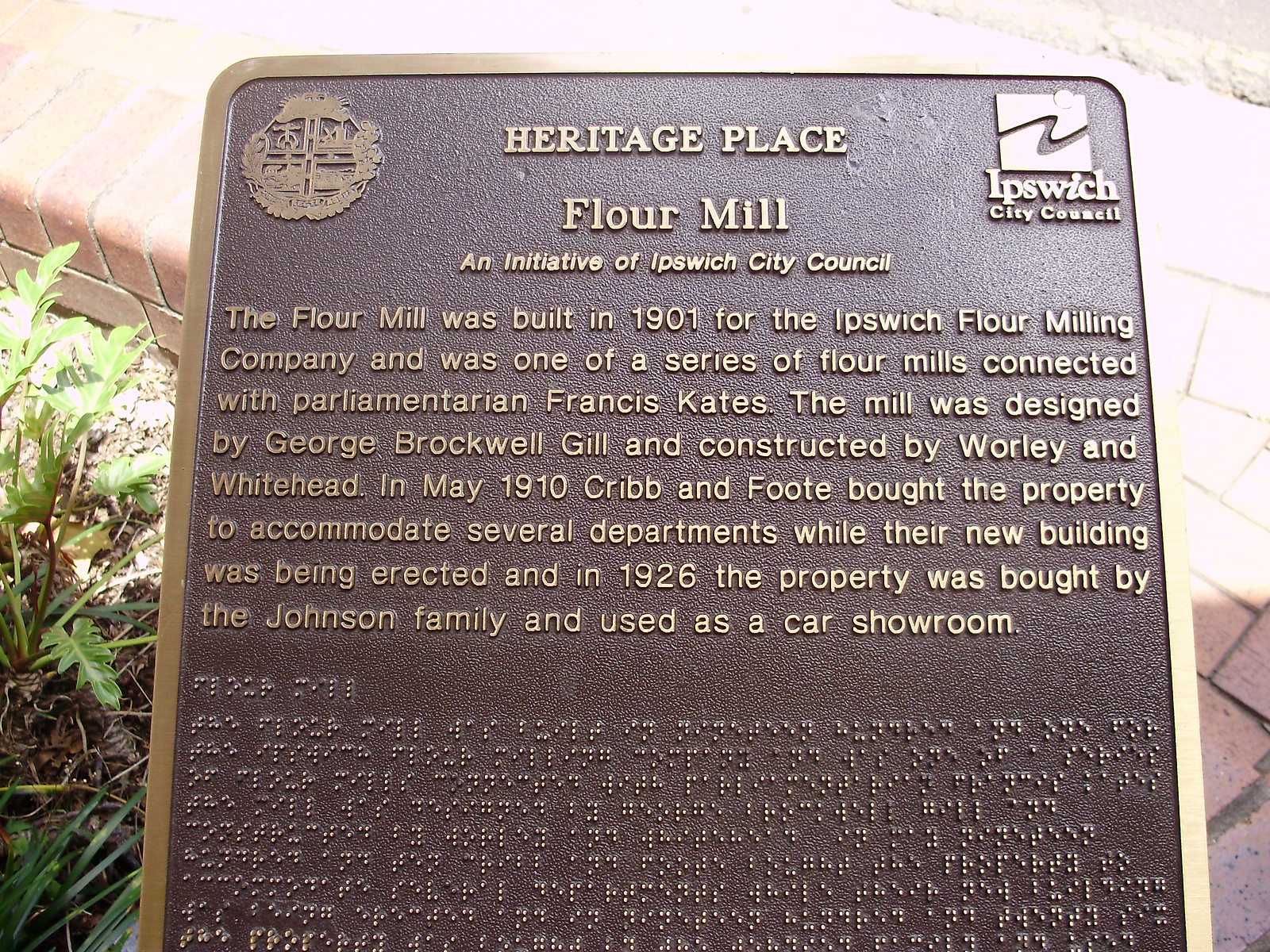This photograph, taken outdoors, depicts a historical marker with a brownish-bronze metal plaque featuring gold-raised lettering and a gold outline. The sign prominently reads "Heritage Place" followed by "Flour Mill, an initiative of Ipswich City Council." The plaque details that the flour mill was built in 1901 for the Ipswich Flour Milling Company and was one of a series of flour mills associated with Parliamentarian Francis Cates. Designed by George Brockwell Gill and constructed by Worley and Whitehead, the property was purchased by Cribb and Foote in May 1910 to accommodate their departments during the construction of their new building. In 1926, the Johnson family bought the property and repurposed it as a car showroom. The same text is also rendered in Braille beneath the main inscription. The plaque is centrally positioned over a brick walkway bordered by a small raised garden bed on the left, with the Ipswich City Council logo and another seal located in the upper corners of the plaque. The upper part of the image is brightly lit, causing the background details to fade out.